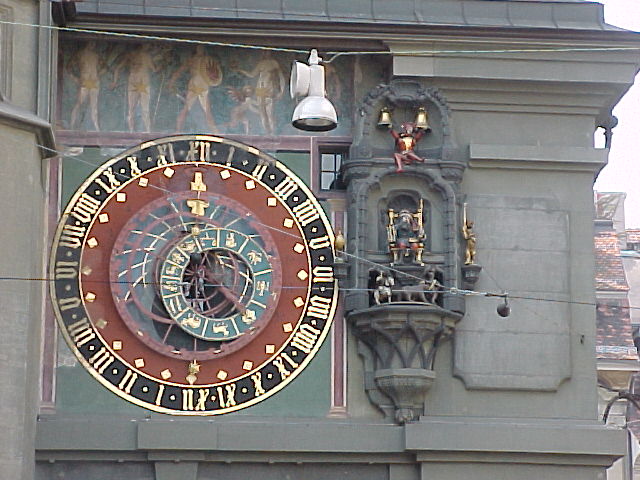This photograph captures the upper portion of a building in remarkable detail, taken from a viewpoint level with the structure but at a distance. On the left side of the image, a prominent clock, which occupies nearly half of the visible section, serves as the focus. The clock is adorned with a golden outline, followed by a black stripe marked with gold numerals. Another gold stripe leads to a dark red segment, within which intricate mechanical gears are visible. Accents of red and white lines surround another inner circle, this one black and embellished with gold symbols.

To the right of the clock, a distinct balcony extends from the building facade. Seated on this balcony is a man in an elaborate throne, exuding an air of regality. Above him, an intriguing figure dressed as a Joker is perched on the building, with its arms seemingly entangled in two bells. This blend of architectural elements and whimsical characters creates a visually captivating scene.